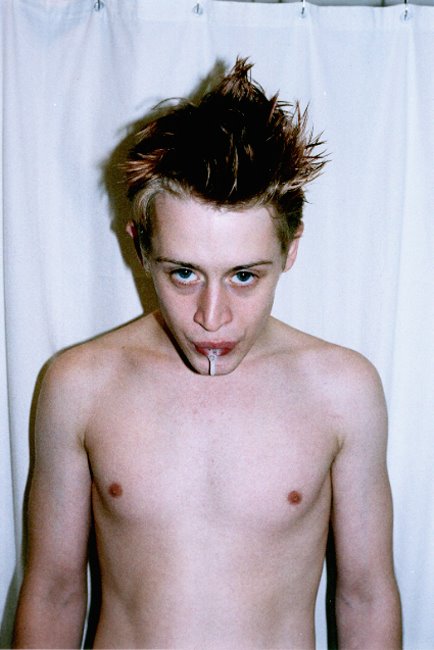This color photograph captures a young, shirtless white male with a striking resemblance to a young Macaulay Culkin. His hair, a mix of dark and blonde hues, appears wild and possibly styled with product. He has very pale skin and blue eyes that lock intensely with the camera. His head is tilted downward while his eyes gaze upward, giving him an annoyed or angry expression. A noticeable detail is the spit or other substance trailing from his mouth, adding to the off-putting nature of the image. Behind him hangs what seems to be a white curtain, likely a shower curtain given the visible rings at the top. The photograph exudes an older, grainy film quality, adding to its unsettling atmosphere.